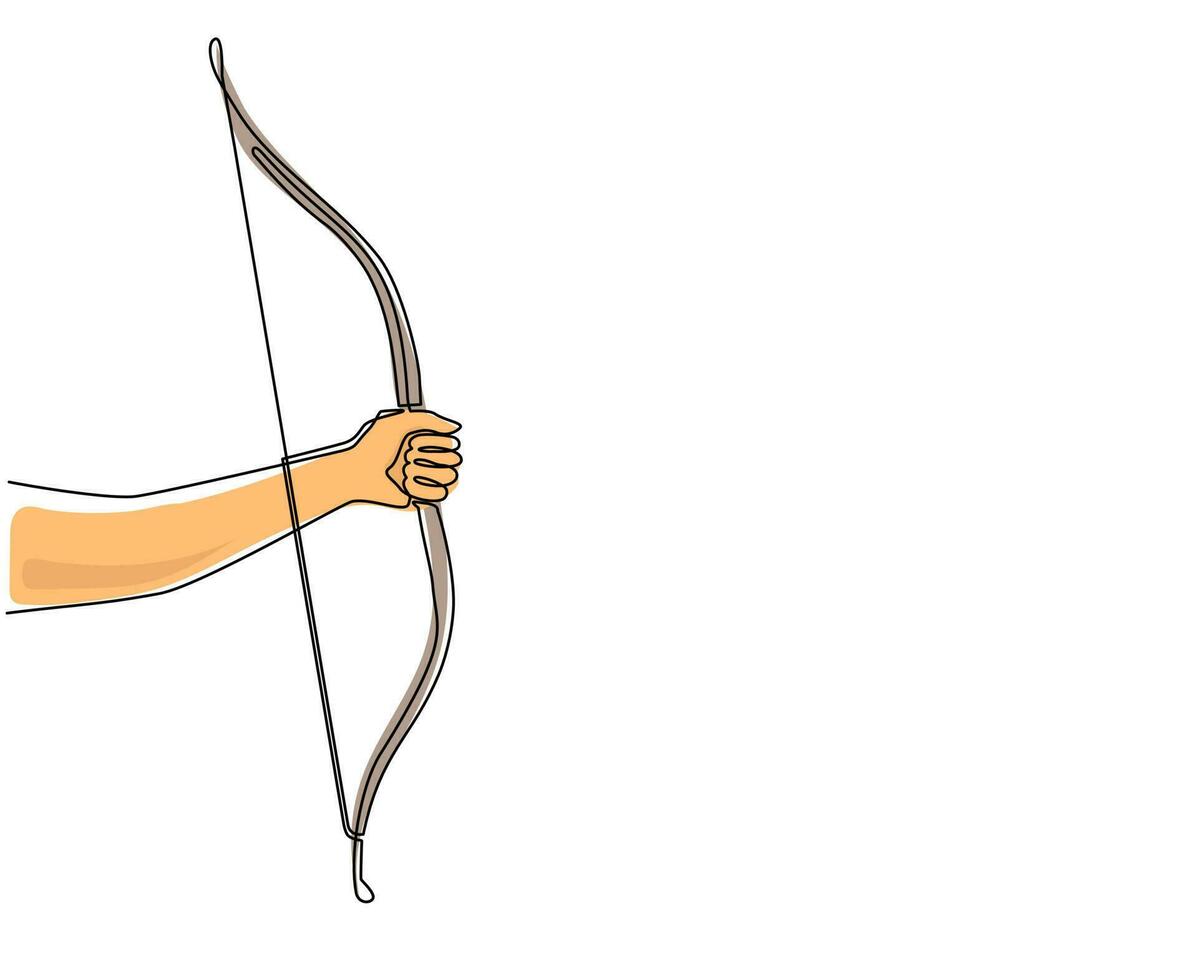This is a detailed photograph of a comic-style illustration featuring the left arm of a person, prominently outlined in black and filled with a light to medium brown flesh tone. The arm, presented with a hand clenched in a fist, extends from the center-left of the frame, reaching out towards the right. The illustration's unique style includes a slight offset between the black outline and the filled color, giving it a distinctive appearance.

The arm holds a vertically positioned bow, rendered in a light brown to gray hue with additional black outlines. The bow's string, a thin black line, runs straight from the top to the bottom of the bow, accentuating its curvature. Subtle highlighting along the top of the arm and throughout the bow adds depth to the image, emphasizing the light brown and slightly darker brown shades within the design. The pure white background further highlights the clean, precise lines and the overall cartoonish style of the illustration.